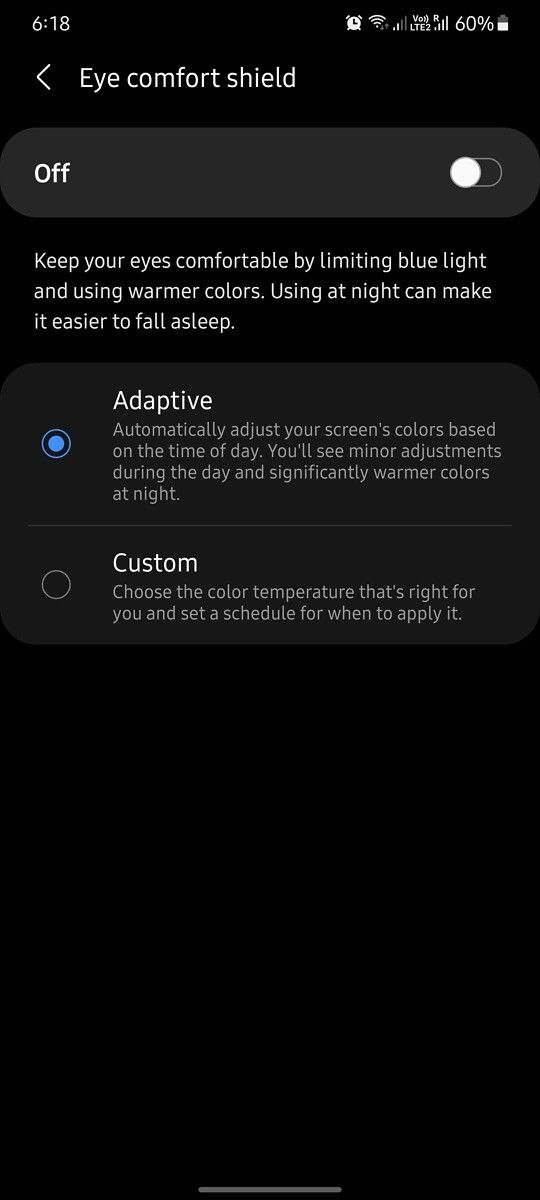Screenshot of Eye Comfort Shield Settings on a Smartphone

The screenshot displays the Eye Comfort Shield settings on a smartphone, and the feature is currently turned off. Eye Comfort Shield is designed to make viewing more comfortable by limiting blue light and using warmer colors, which can help users fall asleep more easily when used at night.

The "Adaptive" mode is highlighted in blue with a blue circle, indicating it is selected. This mode automatically adjusts the screen's colors based on the time of day, making minor adjustments during the day and significantly warming the colors at night for optimal eye comfort.

Below the adaptive mode, there is a "Custom" option which is not currently highlighted. This option allows users to manually choose their preferred color temperature and set a specific schedule for when the Eye Comfort Shield should be active.

At the top left corner of the screenshot, the current time is displayed as 6:18. An alarm symbol is visible next to the time. Additionally, there is a Wi-Fi symbol, an LTE2 indicator, and a battery icon showing 60% charge remaining.